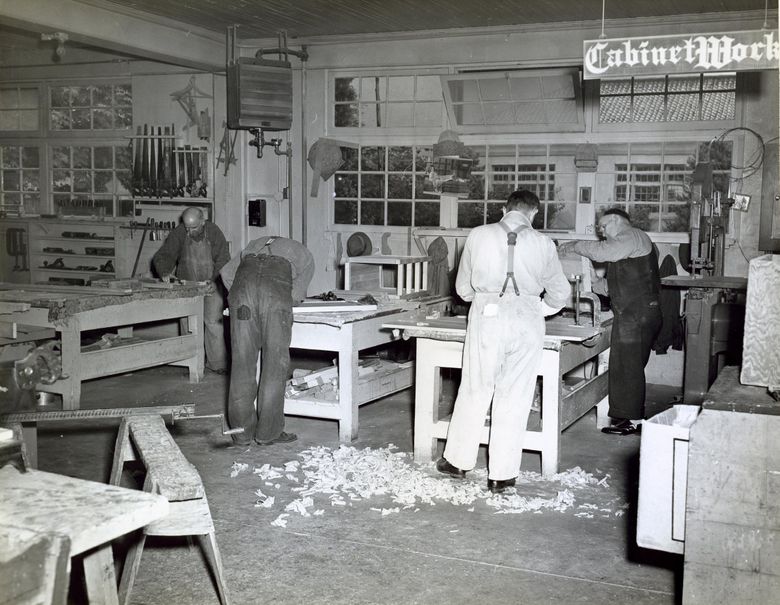This black and white photograph, likely from the early to mid-1900s, captures the detailed interior of an old workshop, potentially a cabinet-making shop. The workspace is defined by large wooden worktables, upon which four men are diligently laboring with various tools and c-clamps. Each of the workers, dressed in baggy jeans, long-sleeve collared shirts, and two with suspenders, are engrossed in their tasks, their bodies obscuring the specific projects they're working on. Black shoes are notably distinct in the grayscale image, with wood shavings or carvings littering the floor beneath them. 

The workshop itself is well-equipped, with tools and pieces of wood adorning the walls, and several windows letting in what little light appears to permeate the otherwise dim space. One window is partially open at the top. To the right, a man wearing a suspended coverall and a shirt stands with his back to the camera, while an older gentleman beside him, donning an apron and glasses, focuses on his work. On the left, another worker, balding, is engaged in an indistinct task, while a fourth man with a patch on his coveralls is bent over, hidden from clear view. Surrounding them are saw horses, benches, a garbage can, and scattered wooden waste, all adding to the authentic, industrious atmosphere of this vintage workshop. High above, a sign that partially reads "cabinet works" hints at the specific nature of their craftsmanship.